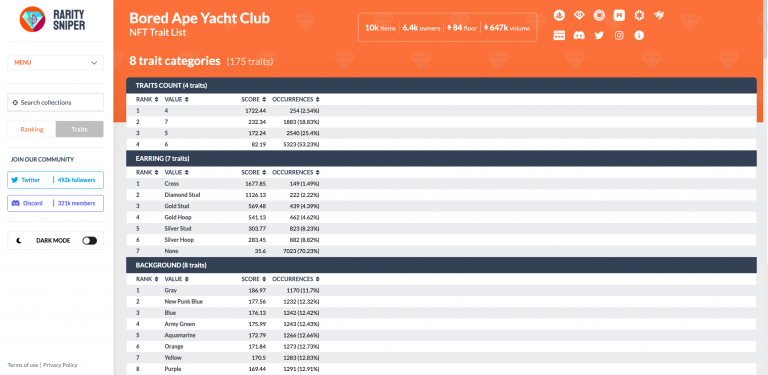This image depicts a detailed interface of the online community for the Bored Ape Yacht Club. The screen features a vibrant orange header at the top, prominently displaying the title "Bored Ape Yacht Club NFT Trait List" in bold white lettering. Directly beneath this header, the interface categorizes information into eight distinct sections, detailing 175 traits, also in white text. 

To the right, vital statistics are noted: "10,000 items," "6,400 owners," "84 floors," and "647,000 volumes," all written in white for clarity. Adjacent to these stats, a series of social media icons are displayed, representing platforms including Discord, Twitter, Instagram, along with several other icons, totaling around ten.

On the left side, a section titled "Rarity Sniper" is highlighted in blue capital letters, accompanied by a blue diamond target icon set within an orange circle. Below this are navigation options for "Menu," "Search Collections," "Ranking," "Traits," and a call-to-action to "Join Our Community." The interface also shows follower counts for Twitter, member counts for Discord, and an option to switch to dark mode.

Further down, detailed trait information is presented, including "trait counts with ranks and values," "earring ranks and values," and "backgrounds with ranks and values," all meticulously listing scores and occurrences. This comprehensive layout offers a robust look into the Bored Ape Yacht Club's digital community and its intricate details.